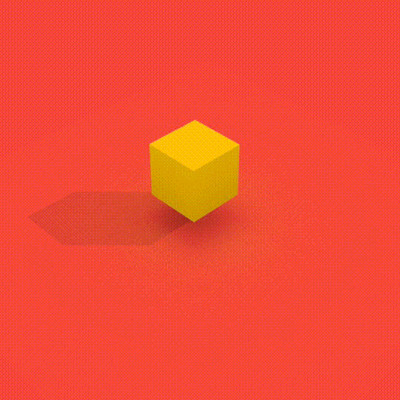This minimalistic digital artwork features a reddish-orange square background with a subtle pinkish gradient. The gradient is darker at the corners and gradually becomes lighter towards the center, evoking a slight orangish hue. Perched slightly off-center within this background is a bright yellow cube, which is balanced on one of its edges. The cube's top face is brightly lit, while the visible sides are shaded in darker yellow tones, emphasizing its three-dimensional form. The intriguing interplay of light and shadow casts a transparent, trapezoid-like shadow to the left of the cube, hinting at a light source from the right and enhancing its geometric appeal. This piece, with its clean lines and elegant simplicity, could make an excellent choice for clip art or artistic background for digital devices.